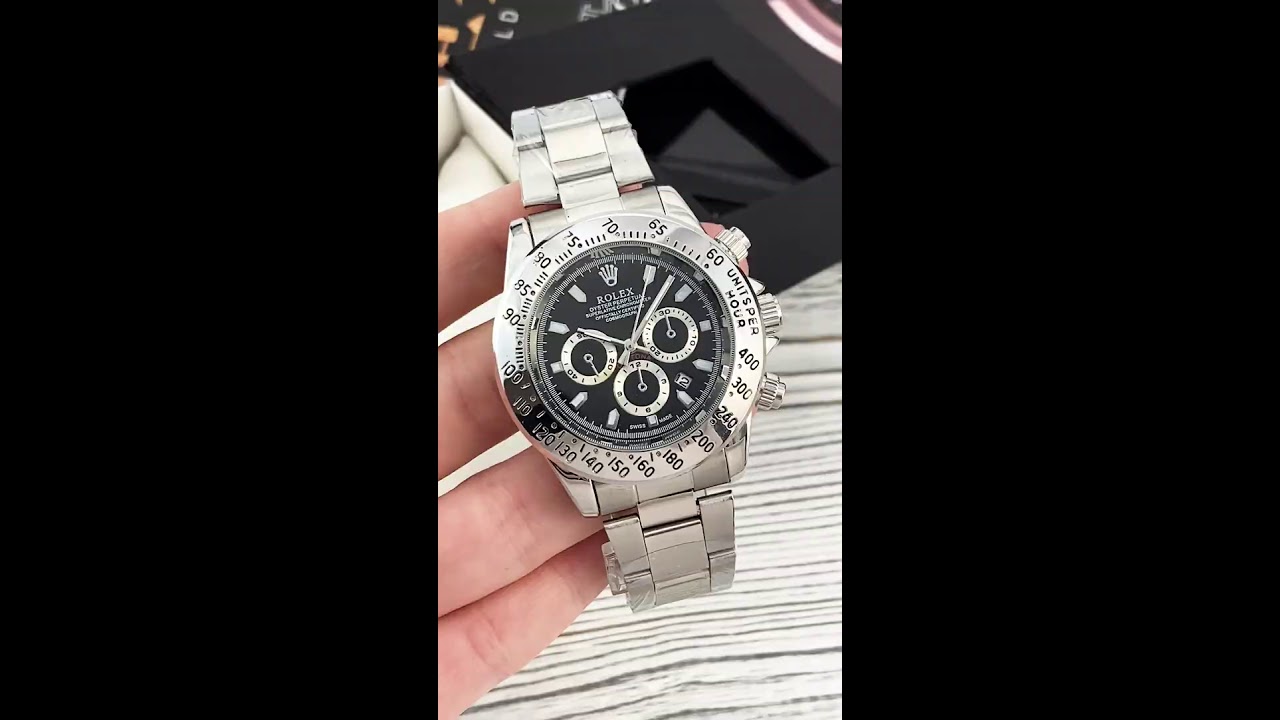In the image, a gleaming silver Rolex chronograph-style watch is prominently displayed, held up close by four fingers of a person's hand coming in from the left side. The watch exudes sophistication with its black watch face adorned by a small crown symbol and the label "Rolex" underneath. The face of the watch also features three small internal chronograph dials and an array of intricate numbers: 60, 400, 300, 240, 200, 180, 160, 150, 140, 131, 20, 120, 10, 190, 85, 90, 75, 70, 65, indicating various time measurements or units per hour. The background of the watch is a combination of black on the upper section and a striped white and gray pattern on a table below. The photograph is presented in a triptych format, with plain black panels on the left and right sides, and the central panel featuring the watch. A mixture of subtle colors, including black, yellow, and orange, can be seen faintly in the background, providing a contrast that highlights the watch’s metallic sheen and immaculate design. Overall, the image conveys a sense of luxury and precision, making the Rolex watch appear exceptionally elegant and desirable.